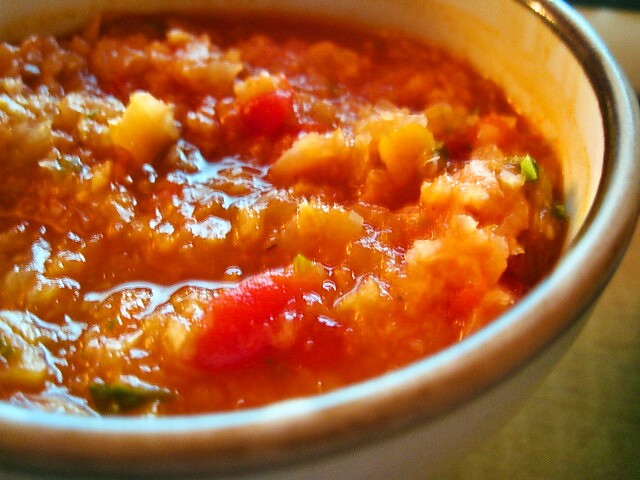The rectangular image is a close-up photograph primarily featuring a heavy stoneware bowl. The bowl, occupying about 98% of the frame, is white both inside and outside, with a distinctive brown trim around its lip. Resting on an off-white surface, the bowl contains a chunky, red, homemade salsa, with a variety of colorful ingredients. The salsa is roughly chopped, brimming with tomatoes, peppers, and flecks of green cilantro, though the pieces are not uniformly cut. Some orange and yellow bits, possibly fruits, add to the visual and flavor complexity. The texture appears thick and slightly mushy, with small, clumpy chunks suggesting elements like potatoes or other solid ingredients. The photograph also shows slight glare and hints of liquid reflection, indicating the salsa’s liquidy consistency. The bowl's inner surface even shows some staining from the vibrant red sauce.